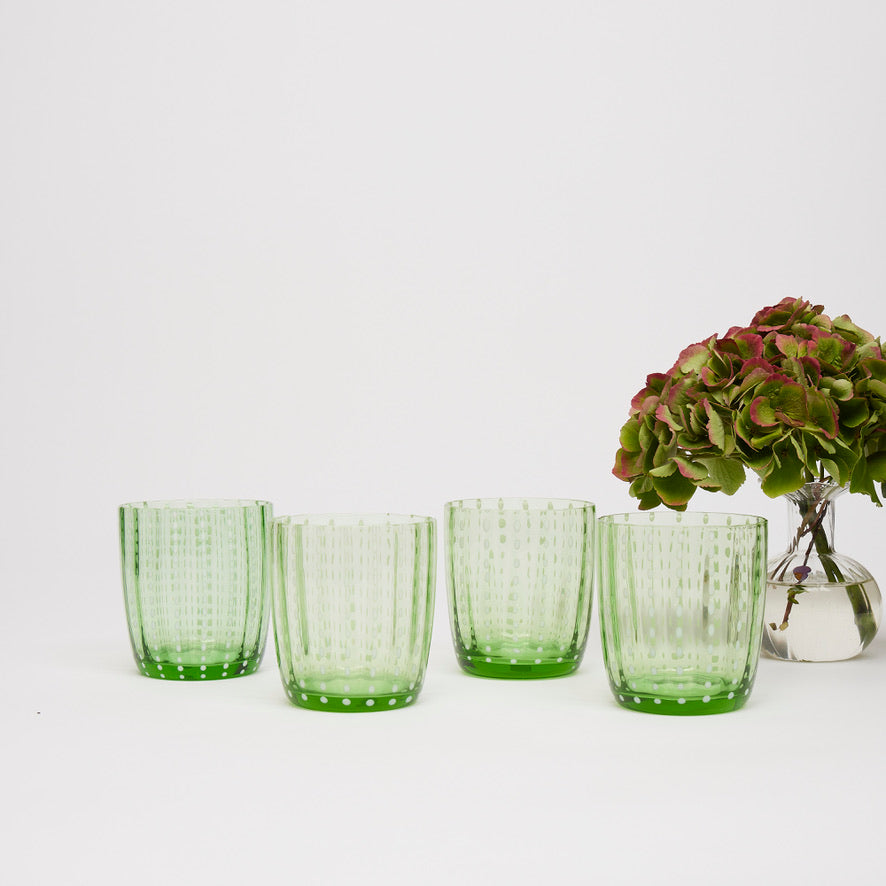The photograph depicts a carefully arranged set of four light green, transparent drinking glasses, adorned with a white polka dot pattern. The glasses are of the tumbler type, short and stout, suitable for serving cocktails or soft drinks. The base of each glass is a slightly darker green, gradually becoming lighter towards the top. Positioned to the right of the glasses is a clear vase filled with water. The vase features a broad, rounded base that tapers gracefully into a narrow neck, reminiscent of a bottle. Emerging from the vase is a plant with densely packed, shrub-like green leaves. The leaf tips exhibit a subtle purplish-red hue along the perimeter. Set against a clean white backdrop, the image captures a harmonious blend of transparency and color, highlighting the detail and texture of both the glasses and the plant arrangement.